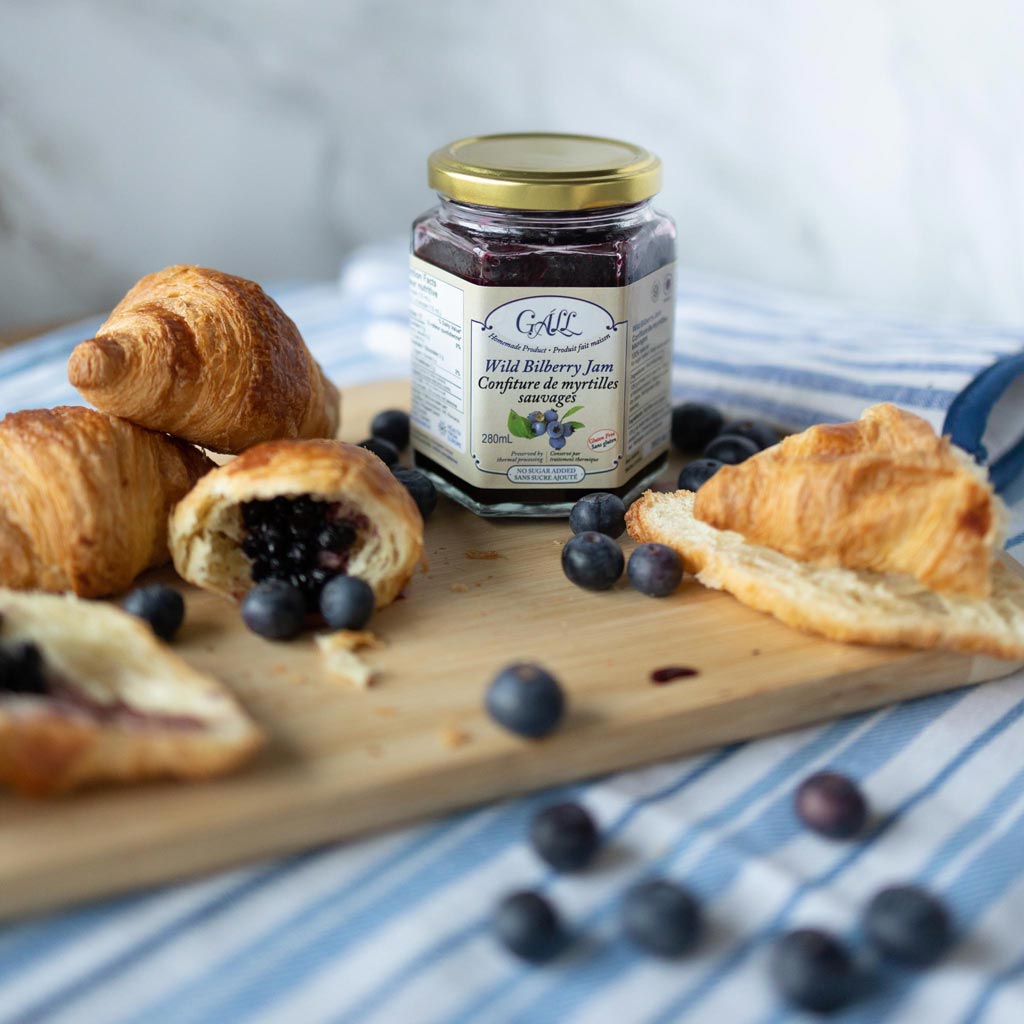The image captures a delightful breakfast spread, meticulously arranged on a blue and white striped tablecloth. Centered on the table is a light wood cutting board, showcasing freshly baked croissants that have a golden-brown, buttery crust. Some croissants are sliced open, revealing their filling of rich Wild Bilberry Jam, while others are stacked neatly. Scattered around the croissants and the cutting board are fresh bilberries that resemble blueberries. In the back corner of the cutting board sits a small jar of Wild Bilberry Jam, identifiable by its gold, hexagon-shaped lid and a label featuring bilberries and green leaves. This charming composition of pastries, vibrant bilberries, and the rustic jam jar evokes a warm, inviting breakfast scene.